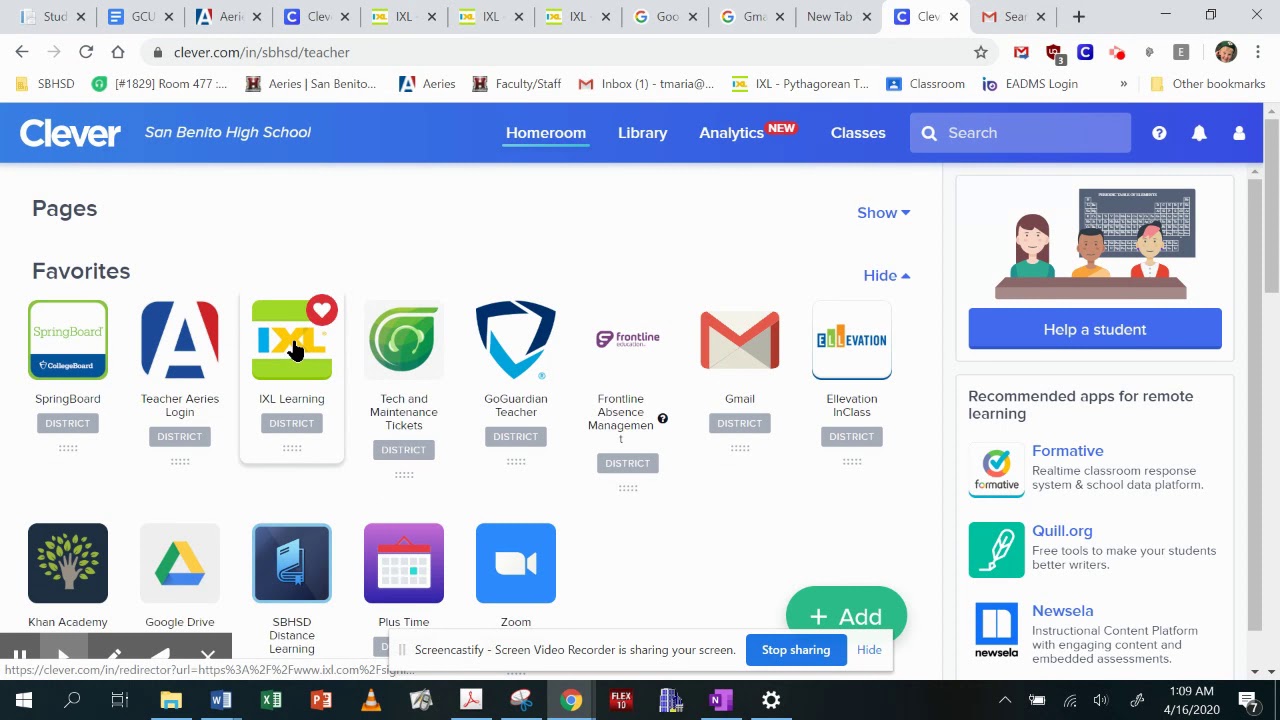In the image, a Chrome browser window is open on a computer running a Windows operating system, as evidenced by the taskbar visible at the bottom of the screen. The user is currently on the penultimate tab, which displays the Clever.com website; this platform is tailored for classroom, teacher, and student use. Specifically, it is customized for San Benito High School. Various educational resources are accessible through this platform, such as Springboard, IXL Learning, and Khan Academy, though the text is slightly hard to read.

The top of the webpage features a blue navigation bar containing links to Homeroom, Library, Analytics, and Classes, alongside a search bar. A separate pane on the right side of the screen displays a cartoon-like image with the text "Help a student," and an associated button. Below this, the section titled "Recommended Apps for Remote Learning" showcases platforms like Formative, Quill.org, and Newsela.